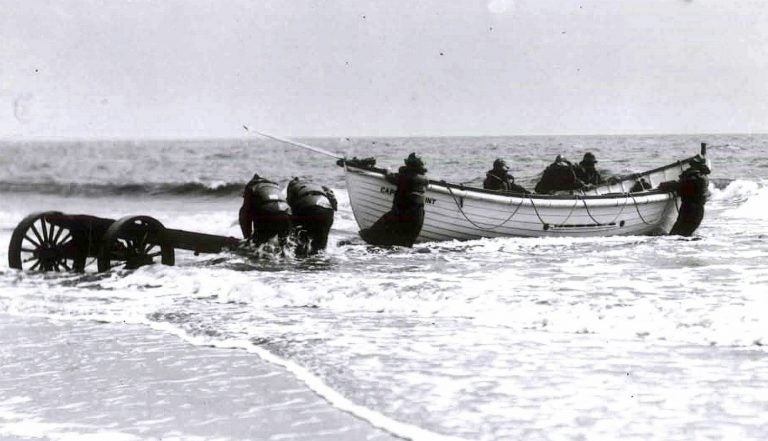This black and white photograph appears to be from a bygone era, possibly around World War One. The image captures an outdoor ocean scene during the daytime. The setting is a beach with foamy waves rolling in and a gray sky overhead. A small boat, seemingly capable of holding around seven or eight men, is central to the composition. The boat, bearing partially visible letters "CAP...NT" on its hull, is being maneuvered by three men inside, while two other men in long black coats are in the water attempting to push it further into the surf. Additionally, two more men are seen bending over a two-wheeled vehicle, likely the trailer used to transport the boat, attempting to maintain their balance in the surf. On the far left, what looks like a cannon or a similar wheeled apparatus is being handled by two men struggling to move it. The overall scene reflects the strenuous effort and coordination among the men to manage both the boat and the equipment in the challenging environment.